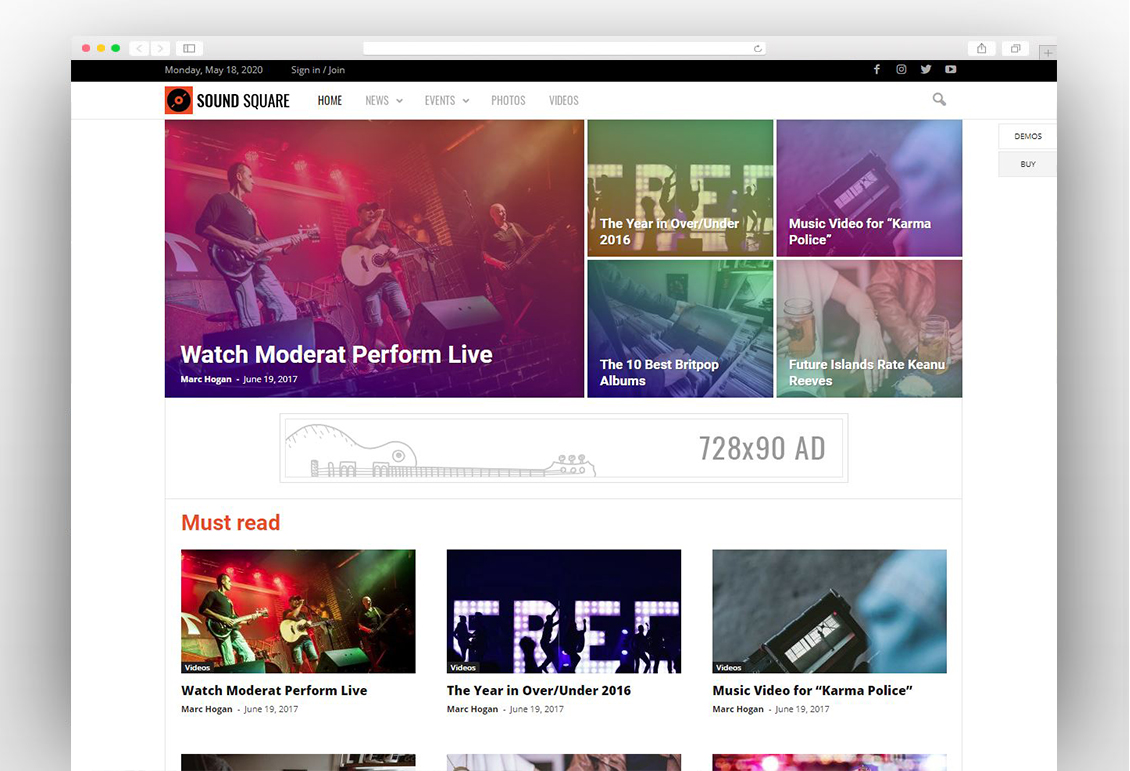This screenshot showcases the homepage of a website called SoundSquare, as indicated by the logo situated at the top left corner. The majority of the background is white, with a narrow black strip spanning horizontally across the top and a light gray section above the main content area. Centrally placed at the top is an elongated white search bar. The light gray borders surround the screengrab on the left, top, and right sides.

Directly below the SoundSquare logo, five categories are arranged horizontally. The leftmost and largest section features a background with shades of pink and purple, depicting three band members performing on stage. This section is captioned "Watch Mode Rat perform live."

To the right of this primary category, four smaller sections are labeled as follows: "The Year and Over Under," "Music Video for Karma Police," "The Ten Best Britpop Albums," and "Future Islands, Ray Keanu Reeves." Situated below these categories, a placeholder labeled "728X90AD" is displayed in gray.

Further down the page, a header in bright orange reads "Must Read," followed by three smaller video thumbnails with black text captions. These videos are titled "Watch Mode Rat perform live," "The Year and Over Under, 2016," and "Music Video for Karma Police."